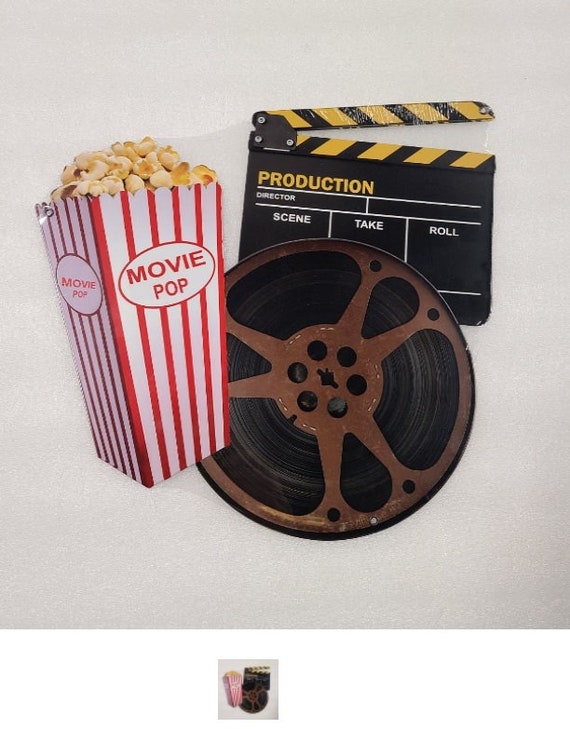This image depicts a collection of vintage movie-themed items against a light gray background, slightly darkening at the bottom right corner. Prominently featured on the left is a classic red and white striped popcorn box, labeled "Movie Pop" in red text within a white circle on both the front and side. Popcorn overflows from the top of the box. To its right, there's an old-fashioned, rusted brown film reel wound with black film. Above the reel is a black clapperboard, marked with yellow and black stripes and the word “Production” in yellow, positioned as if ready to snap. This arrangement, reminiscent of pop art, evokes a sense of nostalgic cinema decor, akin to wall art you might find in a movie theater.